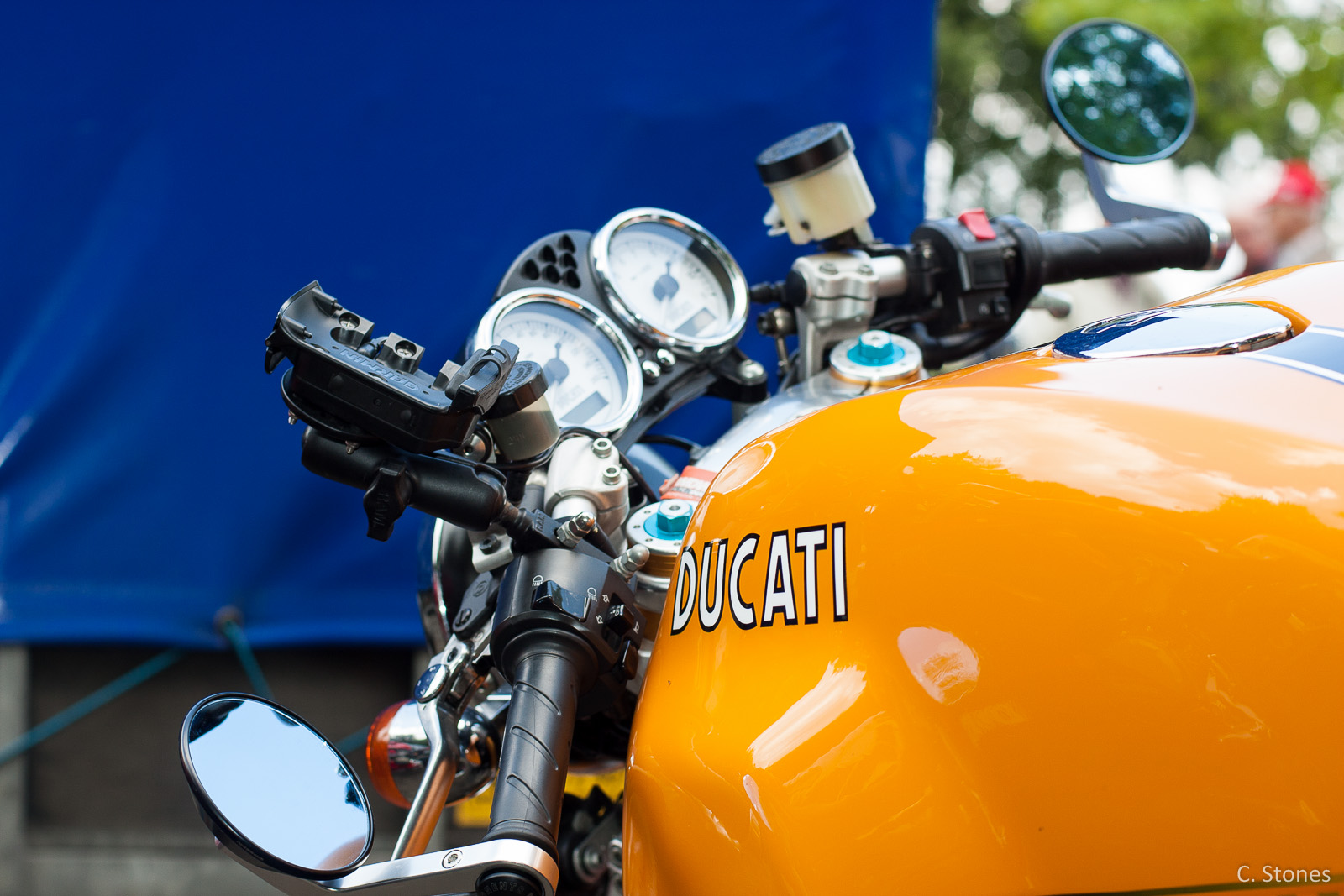The photograph showcases the front end of a Ducati motorcycle, prominently displaying the brand name in white text with a black border on a yellow front panel. A blue stripe runs through the center of the motorcycle, adding a striking contrast to the design. The bike features black handlebars equipped with silver brakes and silver bars attached to round black mirrors. The handlebars also support a phone holder in the center, with a knob on the right side and a white jar with a black cap. Two gauges, likely indicating speed and engine power, are prominently located in the center. 

In the background, a blue tarp is securely lashed to a concrete wall, partially obscured by some faded trees in the upper right corner. The image has a watermark that says "sea stones" in the bottom right corner. The overall focus is on the detailed front section of the motorcycle, leaving the seat, tires, and other parts out of the frame. The visual clarity diminishes towards the back, where the background elements become less defined.